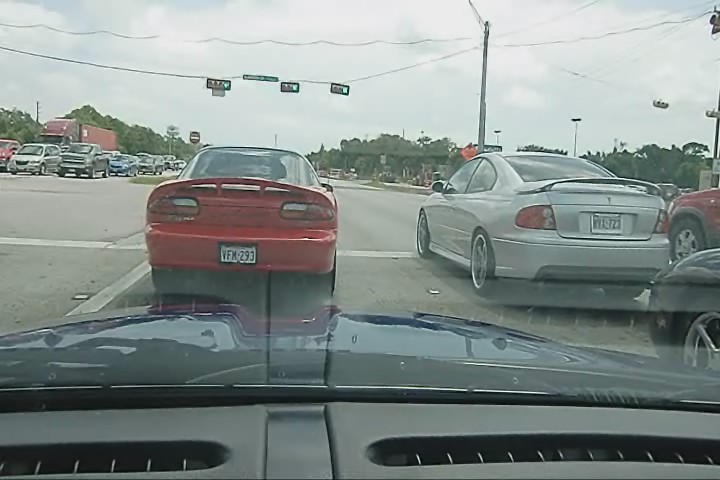This photograph, likely taken with a dash cam or from the dashboard of a car with a dark interior, captures a moment stopped at a traffic light, which has just turned green, on an overcast day. Through the windshield, part of the vehicle’s dark gray hood is visible. In the foreground, there's a row of cars halted at the light. Directly ahead is a red car with a spoiler and a license plate reading VFM 293, and next to it is a silver two-door car, also with a spoiler. To the left, facing the camera, are several other cars. On the right side, you see the front of a black car, and in an adjacent lane is a dark red car. The intersection seems wide with at least three lanes in the direction of travel and additional lanes for opposing traffic seen on the left side of the photo. Traffic lights dangle from overhead wires, and alongside the road are telephone wires, light posts, and commercial buildings with trees in the background. The sky is predominantly cloudy, adding a grayish tone to the scene.